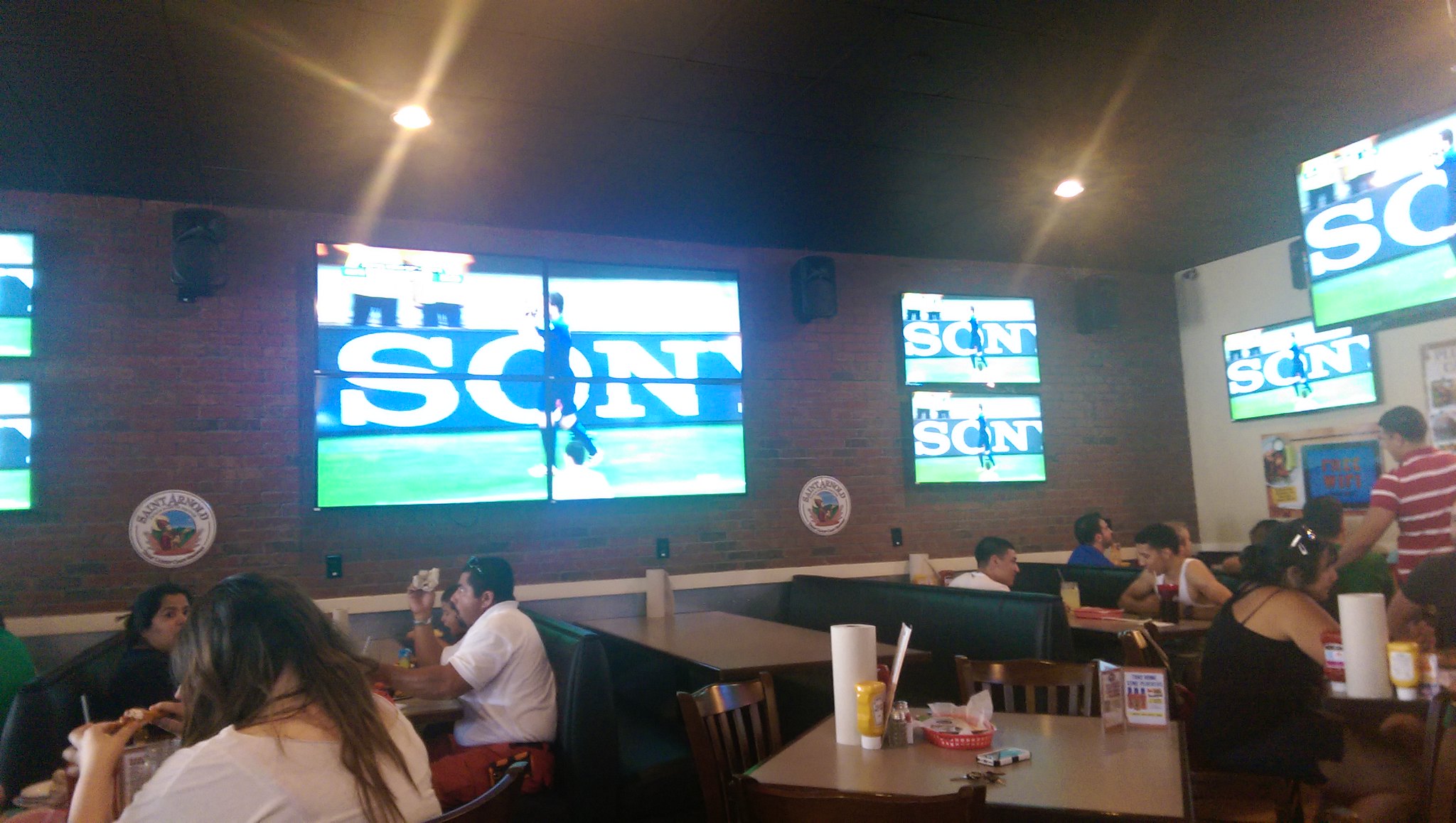This color photograph captures the inside of a casual, family-oriented restaurant that has a distinctive sports bar vibe. The back wall is made of brick and prominently features several large-screen TVs, including a massive one spanning nearly the width of the wall, flanked by smaller screens on either side. Additional TVs are also present on the left side, extending out of the frame. The screens showcase a soccer match with a notable Sony logo visible. The restaurant has a mix of seating options, including brown tables with green booths and brown wooden chairs.

The overall lighting in the restaurant is moderate, giving it a somewhat dim ambiance. The decor is minimal, with functional elements like plastic mustard bottles, rolls of paper towels, and condiment baskets with straws scattered across the tables, indicating a laid-back, cafeteria-style setting. Patrons appear to be diverse in nationality, with some suggesting a Latino or Mexican background, and are casually dressed, wearing white t-shirts, red shorts, black shirts, and one man in a red and white striped shirt standing at a counter. The crowd seems focused on their meals rather than the TVs, contributing to the relaxed atmosphere.